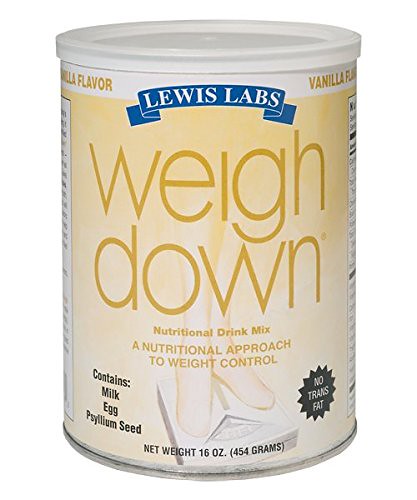This image depicts a cylindrical container of weight loss supplements named "Weigh Down" by Lewis Labs. The container features a prominent white plastic lid, below which there is a blue banner across the top displaying the brand name "Lewis Labs" in white letters. Directly above the banner, yellow text spells out "vanilla flavor," partially visible on both the left and right sides of the label.

The majority of the container's body is orange, fading to a darker orange about a third of the way from the bottom. In the darker orange section, the product name "Weigh Down" is prominently featured. Below this, in smaller, darker brown letters, it reads "Nutritional Drink Mix" and "A Nutritional Approach to Weight Control."

On the bottom left side of the container, black text indicates that the product "contains milk, egg, psyllium seed." Right next to this statement, a white weight scale with the faint outline of feet on it can be seen, further emphasizing the product's focus on weight control. On the right side of the scale, a small black starburst graphic declares "no trans fat." Lastly, at the very bottom edge, the net weight of the product is listed as "16 ounces (454 grams)."